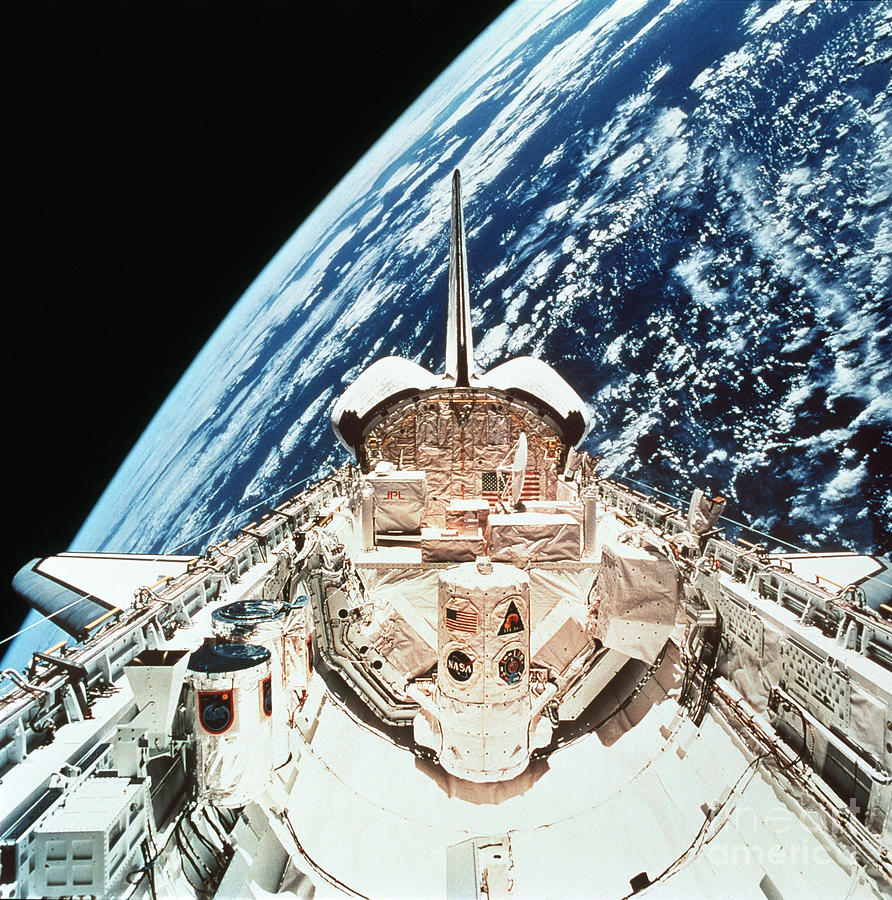The image depicts a large white spacecraft resembling a space shuttle heading towards Earth, prominently showcasing a multitude of details indicative of space exploration. The foreground is dominated by the rear section of the spacecraft, potentially part of the International Space Station, featuring a complex array of components. Central to the image is a prominent cylindrical section wrapped in canvas, adorned with multiple flags, including a small American flag (red, white, and blue) and a circular dark blue NASA emblem with 'NASA' inscribed in bold white capital letters. Additional flags and symbols further embellish this section. The shuttle is equipped with wings and elevated tail fins extending outward, with intricate panels and instrumentation sprawled across its structure. Both sides of the spacecraft exhibit an array of features such as large white barrels with black tops, numerous devices, and visible wiring. The backdrop of the image reveals a stunning view of Earth, highlighting its curvature against the vast expanse of space, with vivid blue oceans, dark expanses, and clusters of white clouds stretching from the upper-right to the lower-left corner.